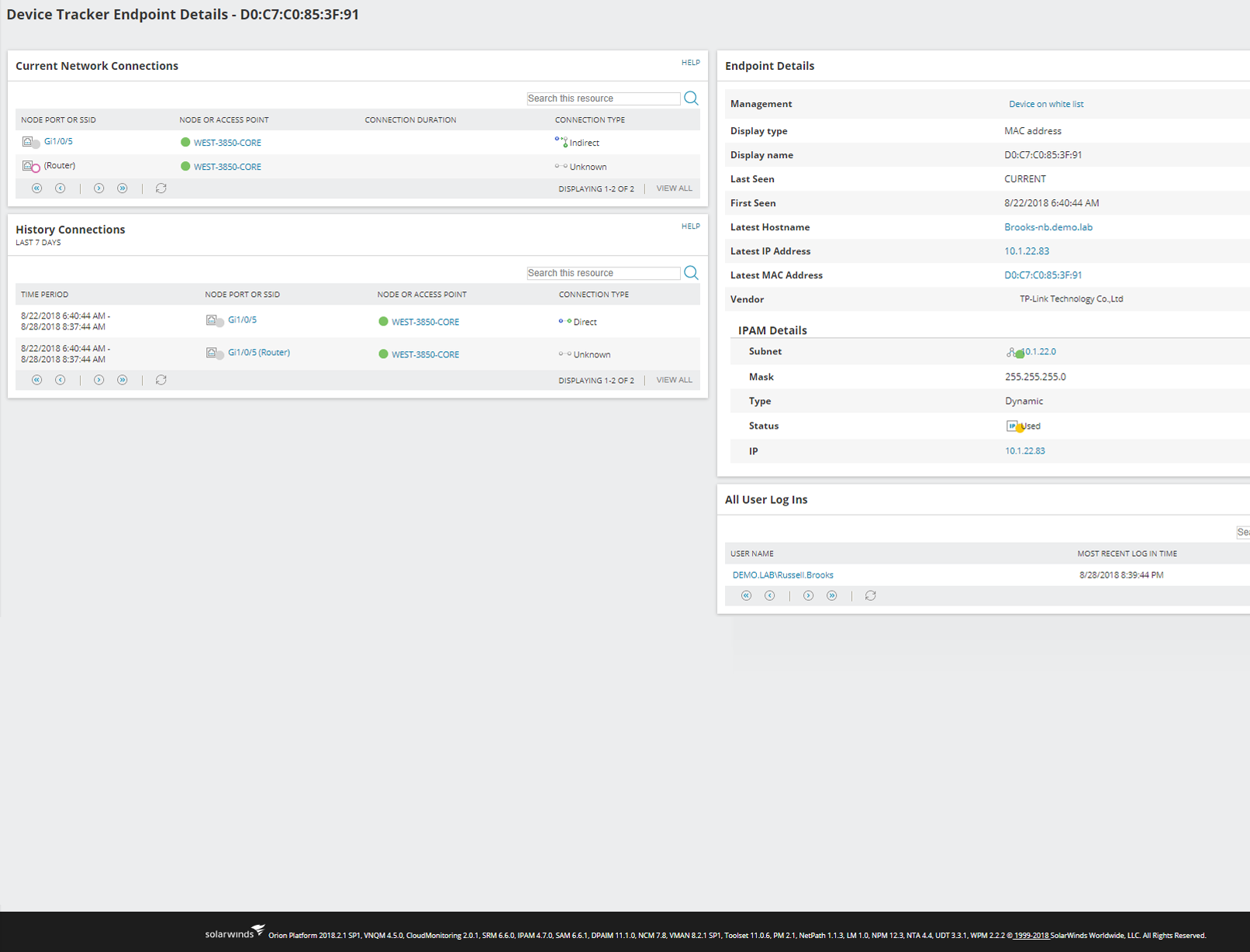Screenshot of a device tracker interface displaying endpoint details. The webpage features a gray background with several white information boxes. At the very top, there's a deal number prominently displayed.

1. **Current Network Connections**: The first white box contains detailed information about the current network connections, represented by various numbers and nearly indistinguishable gray icons. This box includes multiple columns filled out with various types of network data.
   
2. **Connection History**: Positioned below the first box, this section displays a range of historical connection data, again featuring numerous numerical data points and categorized information.

3. **Endpoint Details**: Situated to the right of the first two boxes, this white box is filled with extensive computer jargon, presumably detailing specific endpoint information.

4. **IPAM Details**: The final information box, titled "IPAM Details," is also populated with technical terms related to IP Address Management.

At the bottom of the page, there is a section labeled "All User Logins," which contains various data points related to computer and user login activity.

The overall color scheme and layout present a utilitarian and data-focused interface aimed at providing comprehensive endpoint and network connection details.